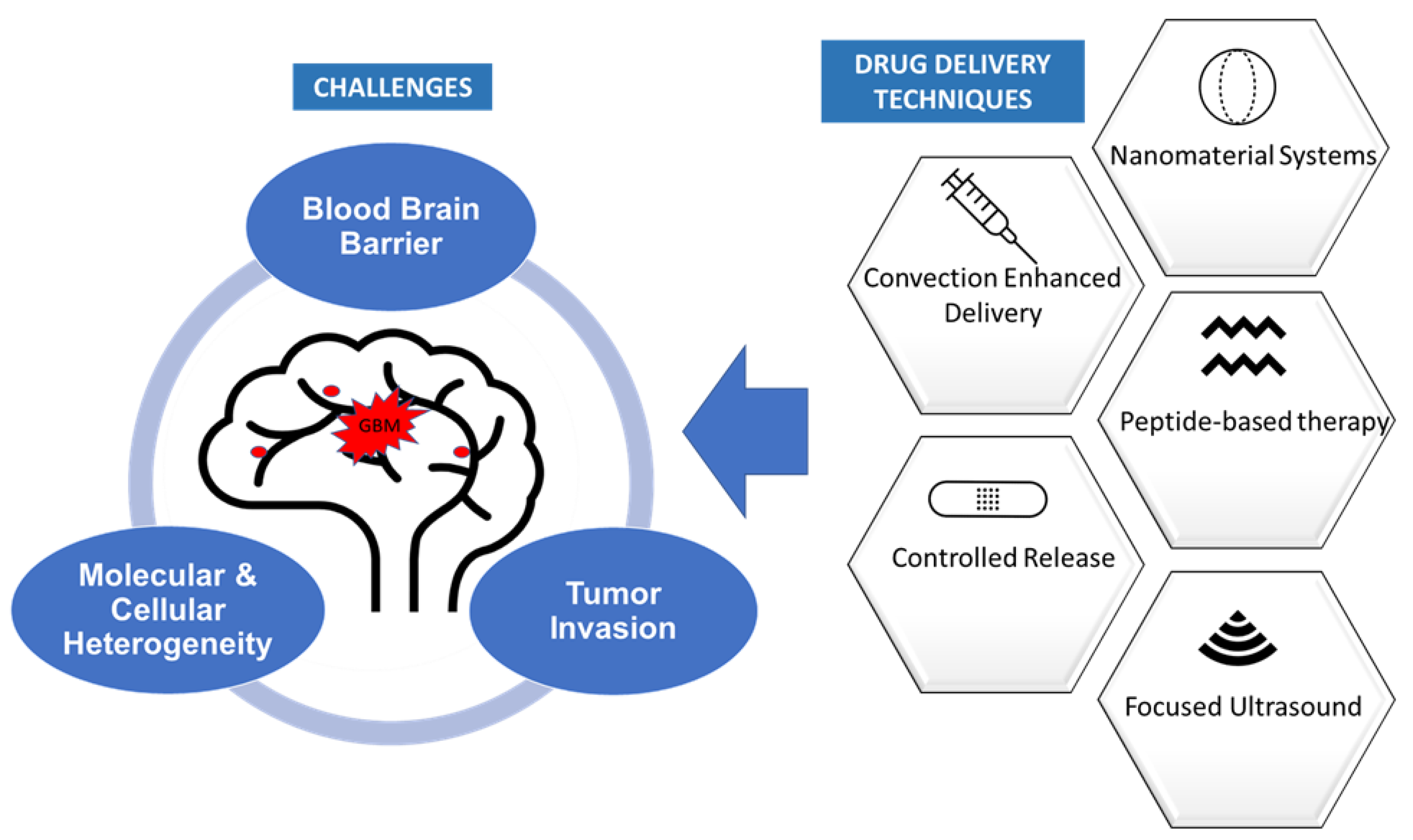The diagram is a detailed flowchart illustrating various drug delivery techniques and associated challenges. On the right side, five pentagon-shaped boxes represent different drug delivery methods: a syringe, a pill, focused ultrasound (depicted with a Wi-Fi symbol), and two others. These boxes are connected by a blue arrow that points to the left. Adjacent to these is a simplified drawing of a brain, set within a blue circle.

Above the brain, a blue rectangle highlighted with white letters labels this section as "Challenges," identifying three major obstacles: the blood-brain barrier, tumor invasion, and molecular and cellular heterogeneity. These challenges are listed within three separate ovals positioned around the brain: the blood-brain barrier on top, tumor invasion at the lower right, and molecular and cellular heterogeneity at the lower left. The right side of the image is also marked by a honeycomb pattern containing the words for each drug delivery technique, emphasizing their distinct categories.

This visually organized flowchart effectively illustrates the complex interplay between drug delivery methods and the significant challenges posed by brain-related treatments.